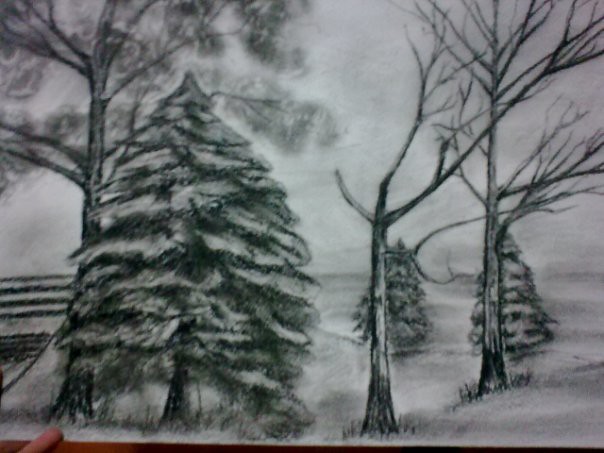The image appears to be a photograph of a detailed pencil or charcoal drawing depicting a serene, wintry scene. The drawing includes several trees, the most prominent being a central fir tree reminiscent of a Christmas tree. To the left of this central fir tree stands a bare tree devoid of leaves, and nearby lies what could be a fence or gate. Further to the right, one can see two more barren trees, with additional fir trees positioned directly behind them, enhancing the forested feel of the scene.

Set against a dark and cloudy sky, the entire scene suggests a cold, bleak winter's day. Some details hint that the ground might be grassy, dusted with what appears to be an artistic representation of snow rather than actual shading. A small roof is faintly visible on the right, oddly positioned as if part of an underground house, blending into the base of a tree. The image includes the tip of a finger pointing towards the drawing from the bottom left corner, suggesting the photo was casually taken without extra lighting. The overall composition lacks text and is rendered entirely in black and white, contributing to its wintry, monochromatic aesthetic.